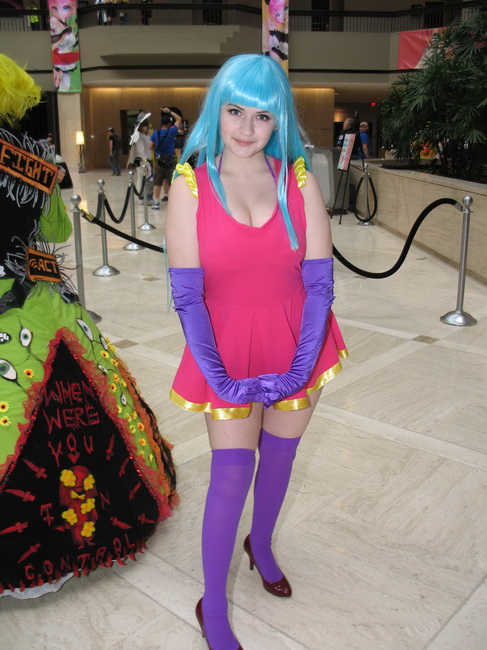The image is a vertically aligned rectangular photograph taken in what appears to be a large indoor area, potentially a mall or convention hall. The floor consists of large square tiles with swirled patterns of beige and light brown. Central to the photograph is a young woman, likely in her mid-twenties, who is dressed up for a cosplay event. She sports a long, straight light blue wig with bangs that partially cover her dark eyebrows. She is smiling up at the camera with her head slightly tilted down. 

Her outfit is a low-cut, sleeveless one-piece dress in hot pink with gold trim, particularly around the shoulders and bottom of the dress. She is also wearing long, elbow-length purple gloves, matching purple thigh-high stockings, and black heeled shoes.

In the background, there are some indistinct, blurry figures suggesting other people are present, fitting for a busy event space. Behind her, there is a roped-off section with steel poles and black ropes, as well as what seems to be a raised area with a tree. To the left of the young woman, part of another person, likely also in cosplay, is visible. This person appears to be wearing a bright green, orange, and black hoop dress decorated with eyeball patterns and a yellow wig. Additionally, there is a partially visible decoration or sign that reads "When were you in control?" in black, yellow, and green colors.